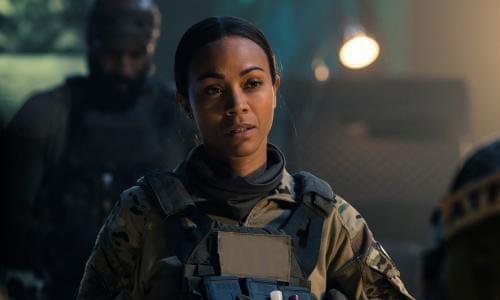In this color photograph, we see a striking, dark-skinned woman dressed in army fatigues and tactical gear, complete with a black bulletproof vest and a backpack. Her dark hair is parted in the middle, falling naturally against her military apparel. She has applied light pink lipstick, and her expression is serious, with her mouth slightly open as she gazes intently at something in front of her. The image captures her from the chest up, highlighting a patch on her jacket and the black tactical straps over her camouflage shirt. 

Behind her stands a man in tactical gear and a helmet, his head bowed, possibly obscuring his face. His blurred presence adds to the intense, somewhat mysterious atmosphere of the photograph. The background is an indistinct mix of dark hues, with one blurry headlamp providing a hint of light but further adding to the overall sense of dimness and tension. The entire scene exudes a sense of readiness and apprehension, typical of a dramatic moment from a television show or movie.